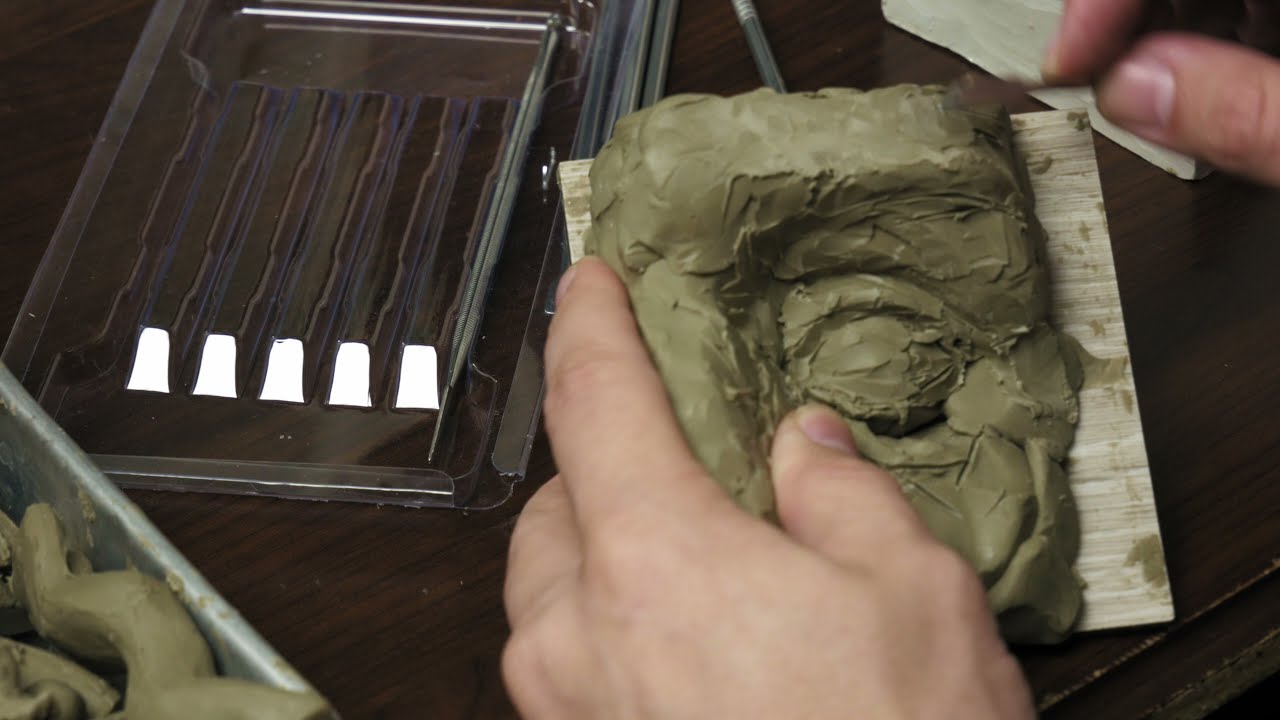In the image, a pair of light-skinned hands are actively working with a piece of dull, grayish-brown clay atop a small wooden board. The left hand stabilizes the board while pressing a thumb into the clay, and the right hand is manipulating a tool to carve small lines and scrapes into the material. Although the clay's shape is undefined, hints of facial features like an eye, nose, and brow can be vaguely discerned in its rough form. The scene is set on a large wooden table that hosts an array of items: a clear plastic tray with several compartments in the top left, a metal tray filled with elongated sticks of green clay in the bottom left, and a variety of metal tools presumably for shaping the clay next to the plastic tray. In the top right corner, an indistinct white object can be faintly seen in the background.